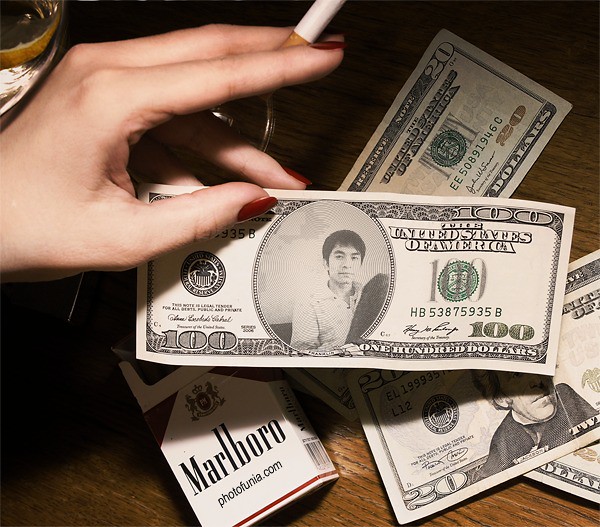In the image, a Caucasian woman's left hand, adorned with red nail polish, is holding a counterfeit $100 bill between her ring finger and thumb. She also clutches a cigarette between her index and middle fingers, with the filter visible at the bottom while the cigarette extends upwards. The counterfeit bill features an Asian gentleman, off-centered, and the phrase "The United States of America," with "the" notably squished. Beneath this fake bill, there are a few $20 bills, which might be genuine, and to the left on a wooden tabletop, there's a pack of Marlboro cigarettes. The cigarette pack has "photofunia.com" printed on it, suggesting the image is an advertisement showcasing the services of PhotoFunia. Additionally, a glass can be seen on the far left side of the image.